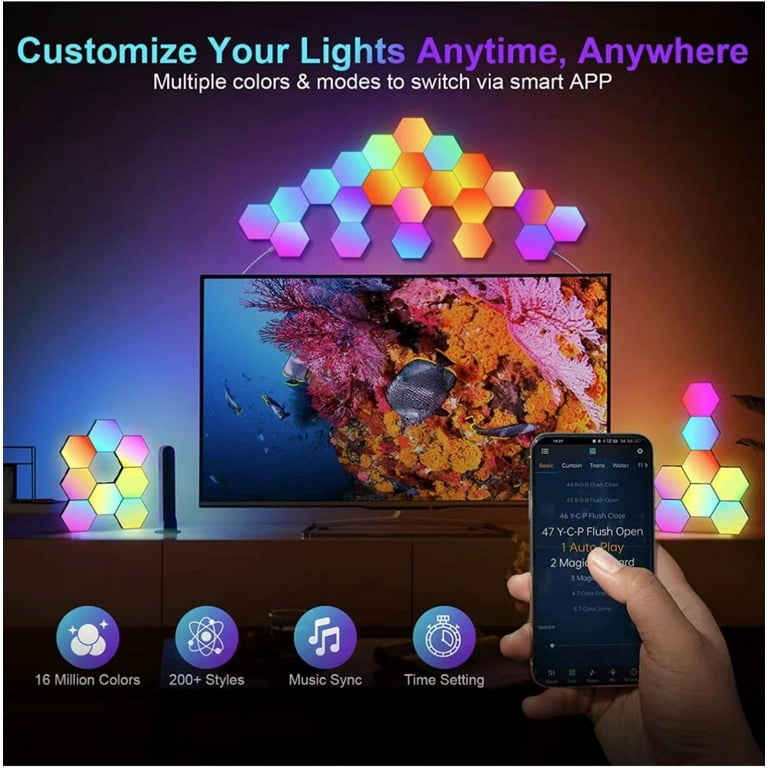The promotional image showcases LED light panels with a detailed view of their functionality. In the foreground, a hand holds a small smartphone displaying an app interface relevant to controlling the LEDs. The screen shows multiple lines of white text, including "46YCP flush close," "47YCP flush open," "autoplay," and other features indicated by circular graphics at the bottom: "16 million colors," "200+ styles," "music sync," and "time setting." The LED panels are creatively arranged in both wall and stand configurations on either side of a television. The top of the image prominently states, "Customize your lights anytime, anywhere, multiple colors and modes to switch via smart app." The lighting in the image includes a variety of colors like light blue, purple, orange, green, pink, and more, highlighting the product's versatility and aesthetic appeal.